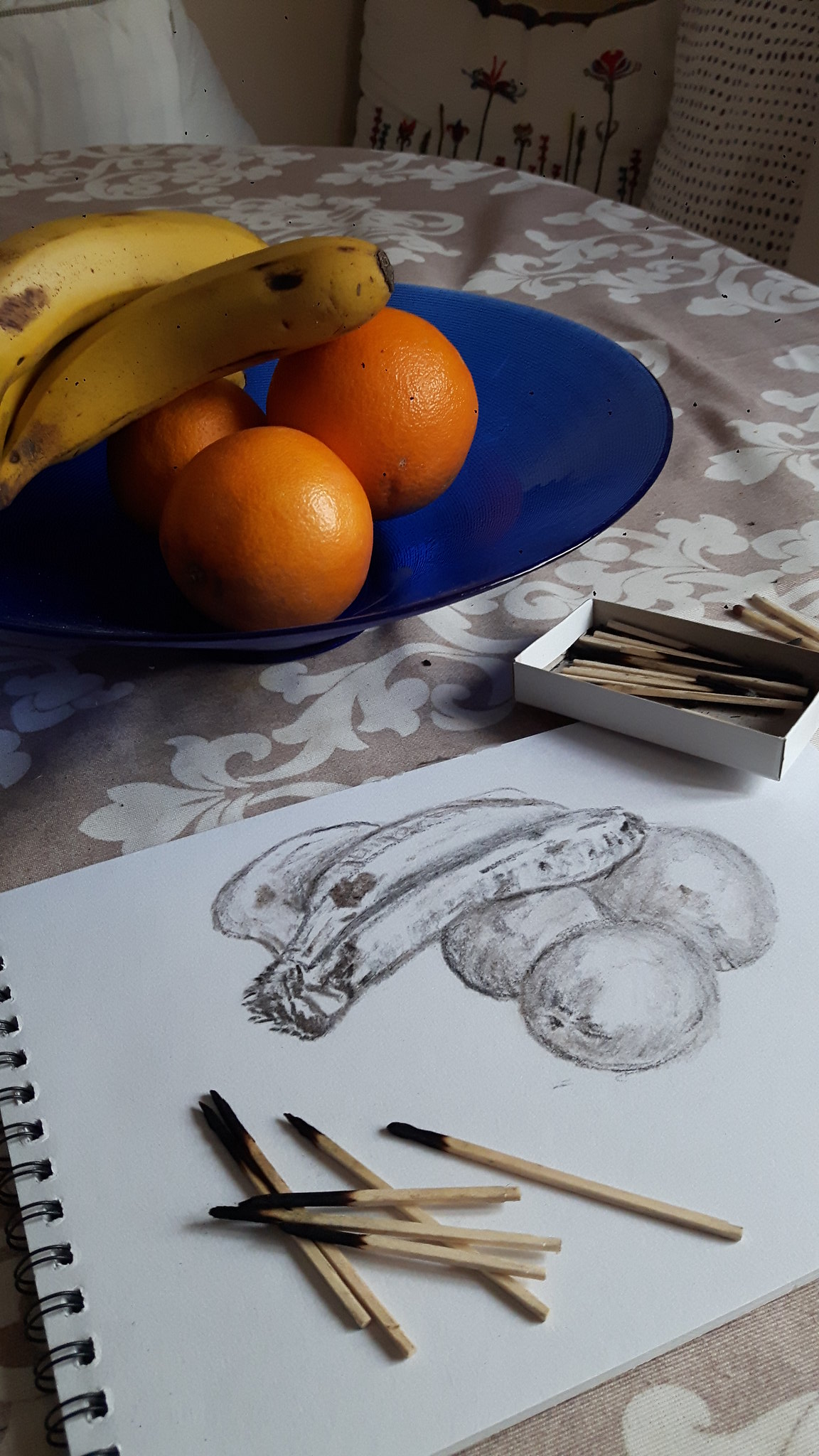This detailed caption describes the intricate scene in the photograph:

"In this captivating photograph of an illustration, the artist has ingeniously used burnt matches to create a drawing that remarkably resembles pencil work. The sketch is displayed on a spiral-bound notebook with pristine white paper. A small pile of burnt matches lies on the paper, hinting at the unique medium used. To the upper right within the illustration, a detailed drawing of a couple of bananas and a few oranges is carefully depicted.

The inspiration for this artistic endeavor is evident in the background, where a blue plate rests on a table covered with a floral white and tan tablecloth in a kitchen setting. On the plate, three oranges and two bananas are arranged, mirroring the subjects of the drawing. Additionally, a matchbox is casually placed on the notebook, further emphasizing the unconventional tools used by the artist. This image captures the creativity and resourcefulness involved in turning everyday materials into a stunning piece of art."